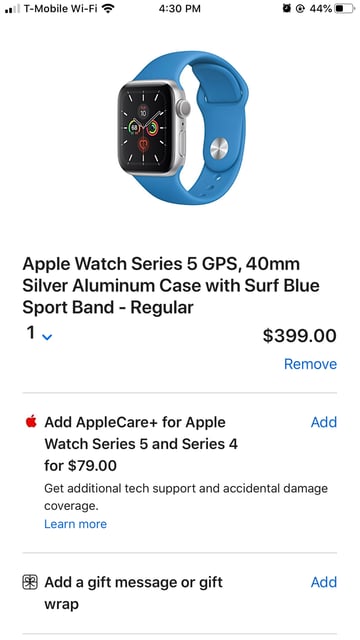This image is a screenshot taken on a phone, showcasing an Apple Watch product. At the top right corner, the phone’s battery status is visible at 44%, represented by a black-filled battery icon. Adjacent to it is an alarm clock icon. In the top middle of the screen, the current time is displayed as 4:30 PM. On the top left, the phone signal strength shows 2 out of 4 bars, and the T-Mobile Wi-Fi signal icon is fully filled, indicating a strong connection.

The focal point in the middle of the screenshot is an image of the Apple Watch. The watch features a blue band with a silver aluminum case, complemented by white arms and dials. Below the image, the product name is detailed as "Apple Watch Series 5 GPS 40mm Silver Aluminum Case with Surf Blue Sport Band - Regular," and it is priced at $399. 

Directly beneath the price, a blue "Remove" option is noted. The bottom half of the image highlights additional purchases: "Add AppleCare+ for Apple Watch Series 5 and Series 4 for $79," accompanied by a blue "Add" button. Below that, there's an option to "Add a gift message," also next to a blue "Add" button.